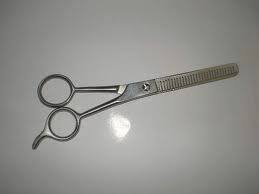The image displays a close-up of a pair of small, steel trimming scissors with blunt tips. The scissors are distinctly silver and slightly reflective, suggesting they are made of stainless steel, though they appear a bit worn. The scissors are laid against a white reflective background, creating noticeable glare and shadows. The design includes two small circular handles; the bottom handle features a small tab extending outward, resembling a comma for thumb or finger placement. Extending from the handles are small metal rods that lead to a central hinge secured by a pin. The hinge allows the two blades to pivot, one of which exhibits a comb-like, filed texture along its edge. The composition suggests the scissors are commonly used for precise tasks like hair trimming or minor surgical procedures. The photograph, albeit a bit blurry, captures the scissors from the lower left to the upper right corner, emphasizing the functional design and reflective surface.